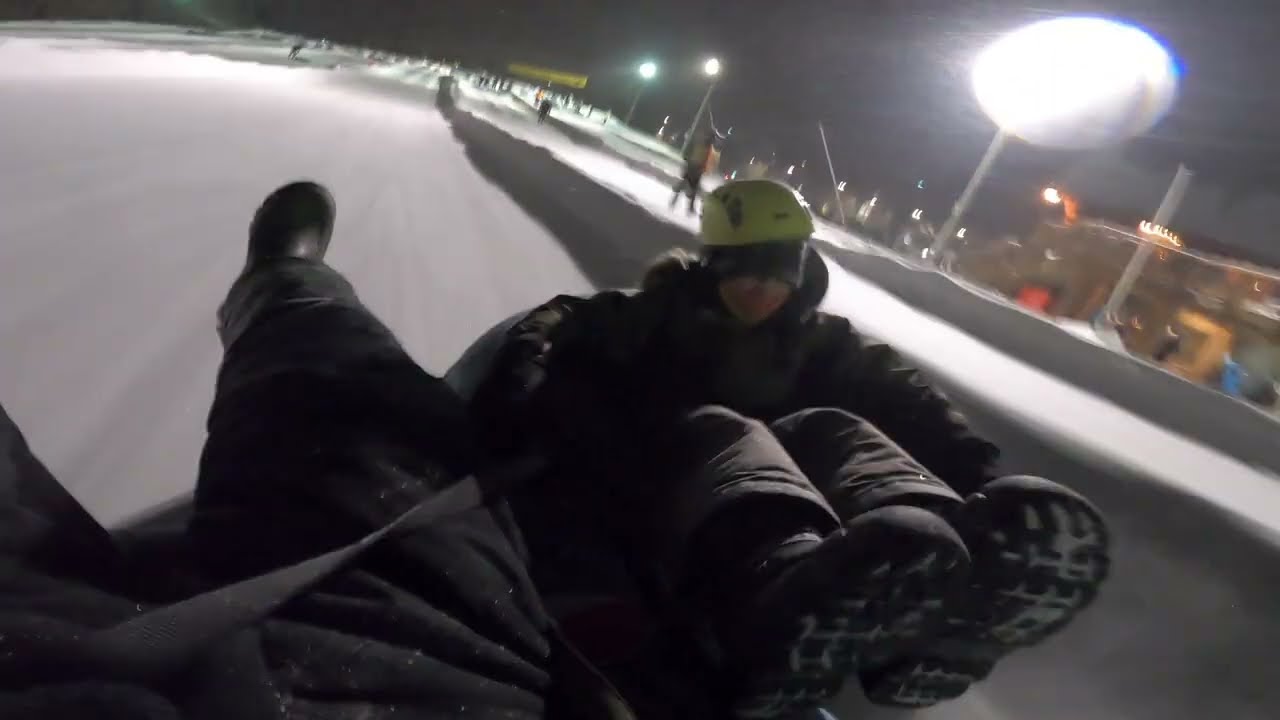In the night sky illuminated by a visible moon, two individuals are seen sliding down a snowy ski slope on a thin black plastic sled. Both are outfitted in black snowshoes, boots, thick pants, and jackets. The person in the forefront sports a neon yellow hard hat over a gray beanie, providing a sharp contrast against their dark attire. Beside them, another figure, only partially visible from the waist down, also dressed in black, accompanies them on the sled. The scene is bustling with distant figures skiing down various marked lanes, indicated by small barriers of snow. Additionally, three lights along the right side of the slope and a blurred building add to the atmosphere, capturing the thrilling winter night adventure.